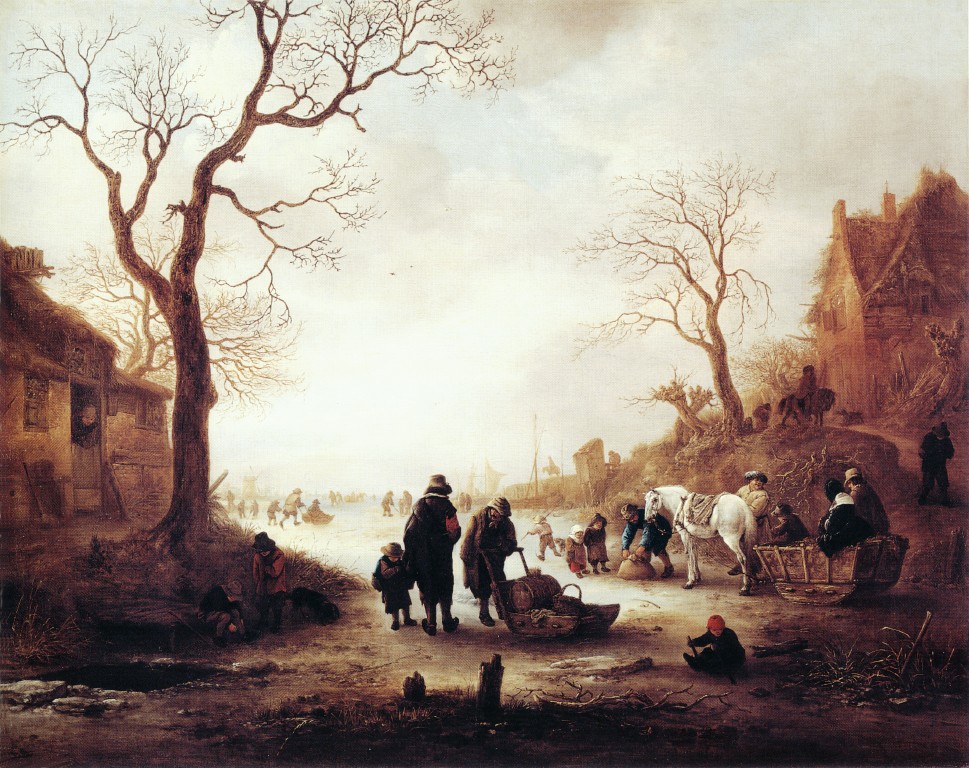The painting appears to be a historical scene, likely set hundreds of years ago, capturing a dreary day in what seems to be a peasant village. The central focus is on a woman pushing a sled with a barrel, flanked on her left by a person carrying a child who is holding their hand, though the child is turned away. To their left, a couple of kids stand in front of a barren tree near a rundown house, where someone peeks out from the doorway. On the right side of the woman, a white horse pulls a sled with a few people on it, heading into the distance, which appears to lead to a body of water, perhaps a lake with a dock. The scene also shows dark figures in the background, suggesting more people on the move, possibly vacating the village. The sky is a muted gray-blue, adding to the overall somber and dreary atmosphere. There are additional barren trees and simple stone houses with thatched roofs, reinforcing the rural setting. A man with a horse and another man running downhill are seen near the house on the right, with more people coming down the path. The limited use of color amidst predominantly muted tones enhances the painting's bleak appearance.